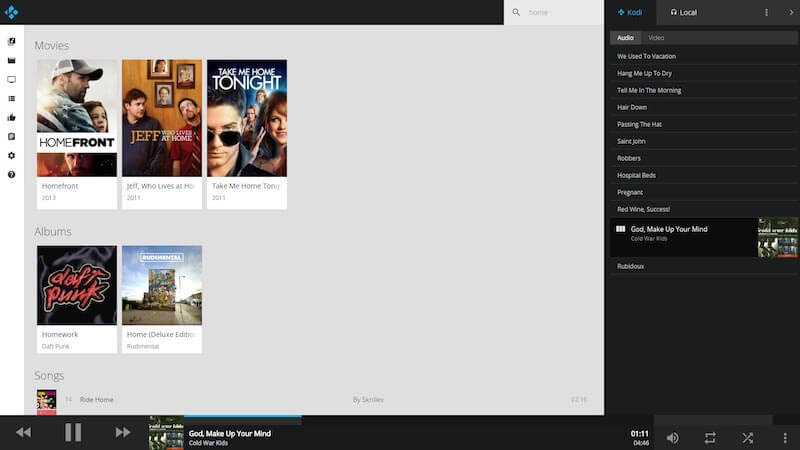The image appears to be a screenshot of a webpage. In the top left corner, there is a diamond-shaped icon divided into four unequal parts, forming the letter "K." In the upper right corner, there is a grey search box with a magnifying glass icon, allowing users to enter text. To the far left, there is a vertical column of icons representing various actions: stacked pages, screens, a thumbs-up, a star, and a circle containing a question mark.

The main body of the webpage features a grey background and showcases five movie titles in a grid format: three titles on the first row and two on the second. The first movie, "Homefront," displays a man wearing a hat holding a young girl, with another man below the title. The second movie, "Jeff Leaves at Home," shows two men sitting down; the man on the left is in a black hoodie, while the man on the right wears a short-sleeve red shirt and a tie. They are looking at each other, with three pictures hanging on the wall behind them. "Take Me Home Tonight," the third movie, features a man in sunglasses on the left, two women in the background, and another woman with red hair in the foreground.

The second row of movies includes "Daft Punk," written in red font against a black background. Below it is an image resembling a mural on the side of a building, with a street light on the left. To the right of this section are various options on a black background. These include audio and video settings, and a list of different song entries such as "We Used to Be on Vacation," "Hang Me Up to Dry," "Tell Me in the Morning," "Her Town," "Passing the Hat," "St. John," "Raycon," "Historical Habits," "Preaking," "Red Wine," "Success," and "God Make Up Your Mind."

Below these options, there are playback controls including forward, pause, and fast-forward, along with the title of the current song, "God Make Up Your Mind." On the far right, additional options are displayed: the current time, speaker settings, shuffle options, and menu access.